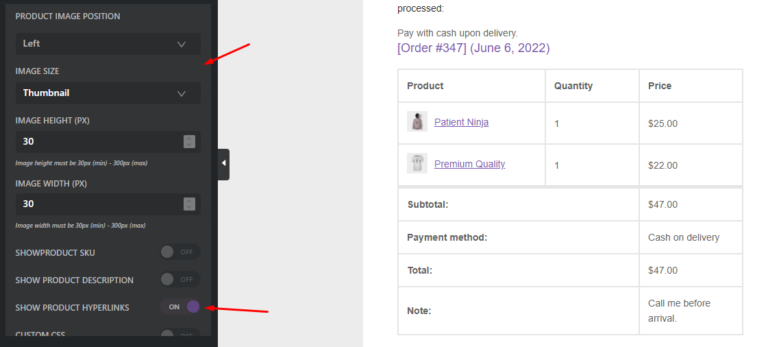A detailed screenshot of a website is displayed, split into two distinct sections. The right half presents an order summary with clear details:

- **Order Number**: 347
- **Date**: June 6, 2022
- **Payment Method**: Cash on Delivery

A tabular column lists the products ordered:
1. **Product**: Patient Ninja
   - **Quantity**: 1
   - **Price**: $25
2. **Product**: Premium Quality
   - **Quantity**: 1
   - **Price**: $22

The order subtotal is $47, matching the total of $47. A notable customer note mentions, "call me before arrival."

The left half reveals the website's settings, featuring a dark grey background contrasting with the overall white theme. The settings include:

- **Product Image Position**: Left
- **Image Size**: Thumbnail
   - **Image Height**: 30 pixels
   - **Image Width**: 30 pixels

Indications of additional settings with red arrows show:
- **Show Product SKU**: Off
- **Show Product Description**: Off
- **Show Product Hyperlinks**: On